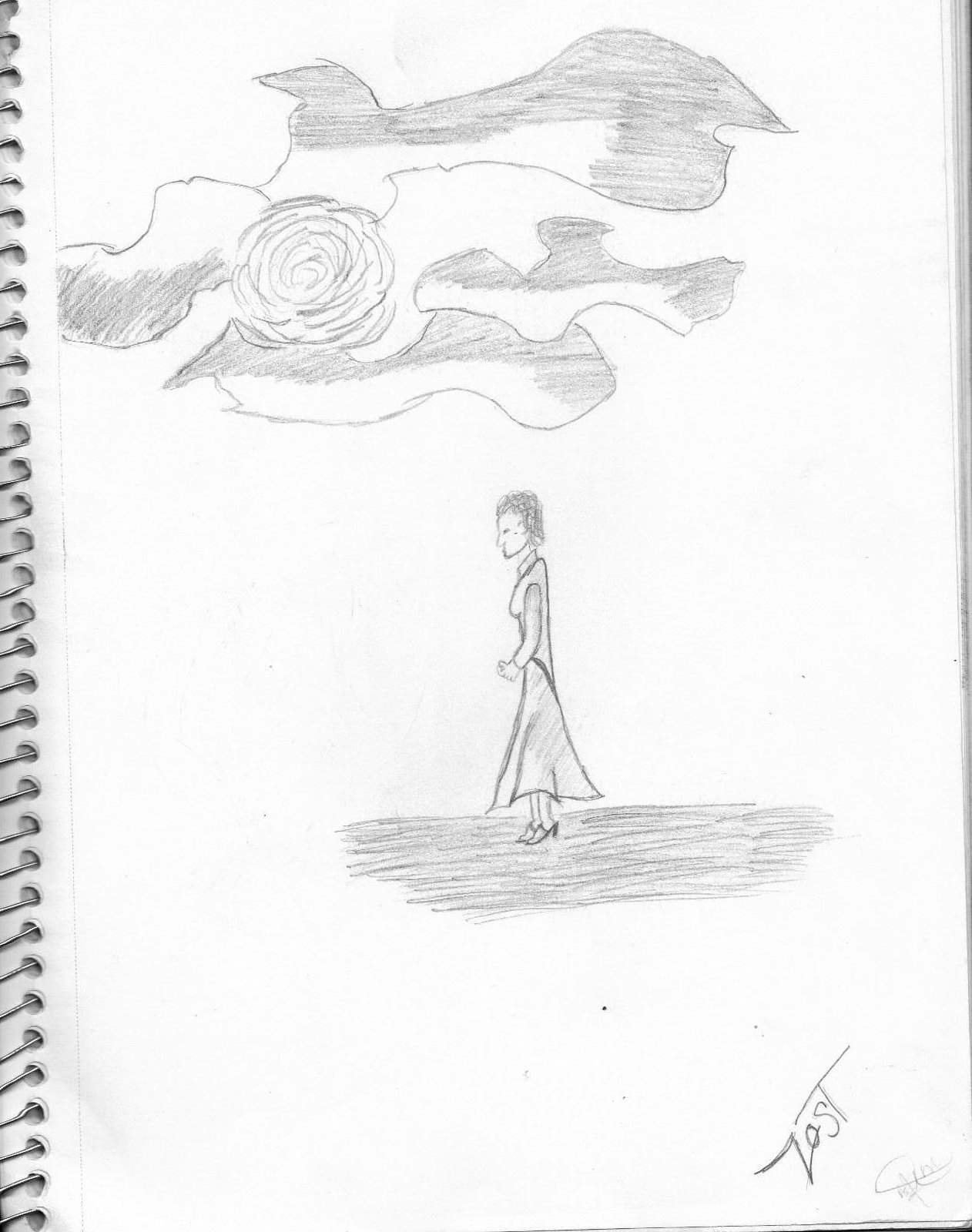A detailed pencil drawing on sketch pad paper, complete with visible ring-binding along the left edge from the scanned image. The focal point of the illustration is an older woman standing on a dark, shaded surface. She is elegantly dressed in a vintage-style dress and high-heeled shoes, with her hand resting by her side. Above the woman, the sky features an ambiguous celestial body that could be interpreted as either the sun or the moon, accompanied by uniquely shaped clouds that are distinctly shaded, appearing half white and half dark. The artist's signature, "ZOST," is elegantly inscribed at the bottom of the image.